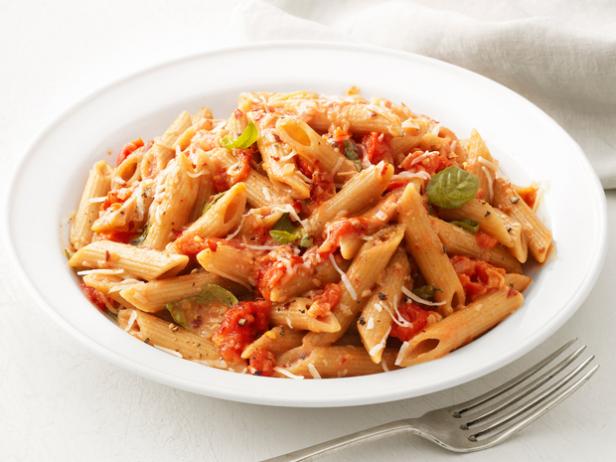This photograph showcases a delicious pasta dish prominently centered on a pristine white tablecloth. The white porcelain plate brims with penne pasta, generously portioned and almost overflowing. Scattered chunks of ripe tomato and random individual green basil leaves adorn the pasta, adding a splash of color and freshness. A light dusting of grated cheese sits delicately atop the dish, enhancing its visual appeal and flavor without overwhelming the ingredients. There’s a faint presence of some kind of spice mixed within the sauce, giving it a subtle complexity. In the lower foreground, a regular silver metal fork is positioned diagonally, suggesting an invitation to indulge. The faint outline of a white cloth napkin can be seen in the upper right corner, adding to the elegant dining setup. The photograph, while not crystal clear, is of good quality and exudes the professionalism of a restaurant menu promotion, emphasizing the appetizing appeal of this freshly made pasta dish.